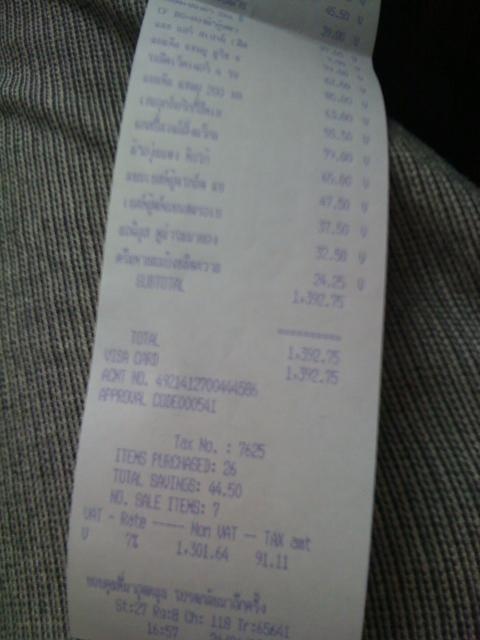This photo captures an out-of-focus, long and narrow white receipt featuring text in a purple-blue typed font. The text appears to be in Thai, suggesting the receipt originates from Thailand. Detailed item descriptions in Thai and corresponding prices are listed on the receipt, with at least eight to ten distinct purchases visible. The total amount, somewhat illegible due to the blur, seems to exceed one thousand units of the local currency. Payment was made using a Visa card, as evidenced by an approval code displayed on the receipt. The receipt also indicates that a total of 26 items were purchased.